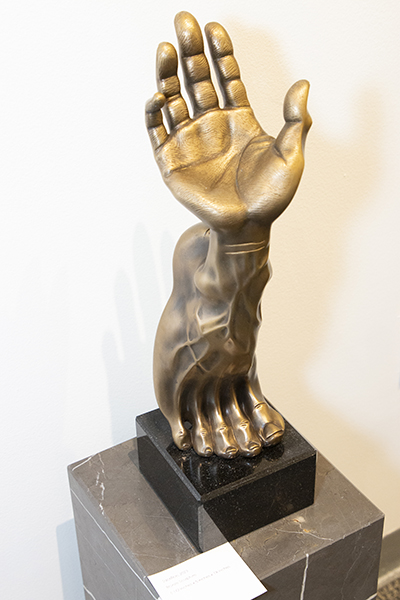This photograph showcases a detailed bronze sculpture, vividly capturing the surreal fusion of a foot and a hand. The sculpture is composed of a hand, palm facing upward, seamlessly transitioning at the wrist into an ankle that extends into a foot poised delicately on its tippy toes. The intricate detailing highlights visible veins in the foot and the individual digits of both the hand and the toes. The sculpture has a goldish-brass color and is prominently displayed on a black marble cube, which itself rests on a larger rectangular pedestal of brown marble with white inclusions, possibly in a gallery setting. A small paper tag is placed atop the pedestal, and the backdrop features a white wall that casts distinct shadows from the sculpture, adding depth to the presentation.